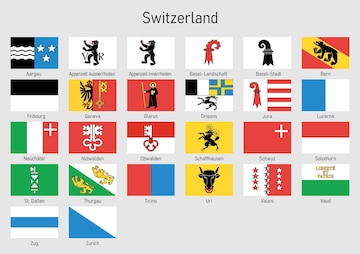The image is a color illustration of Swiss flags, presented in a landscape orientation on a light gray background. At the top, in black text, the title "Switzerland" is prominently displayed. The illustration consists of six flags per row across four rows, with two additional flags on the bottom left, totaling 26 flags. Each flag has a black text label beneath it, indicating the city or region in Switzerland it represents.

The flag designs are diverse, showcasing a range of colors and symbols. Notable examples include a black flag with white waves paired with blue and three stars, several white backgrounds featuring lion sigils, a white flag with a red sigil, a yellow and red flag depicting a bear, and a striking black and white striped flag. Other flags display patterns such as blue and white triangles and red and blue rectangles, and one features a yellow background with a black bull face. The style of the image combines color illustration with text and graphic design elements, though the text descriptions under the flags are blurry and difficult to read.